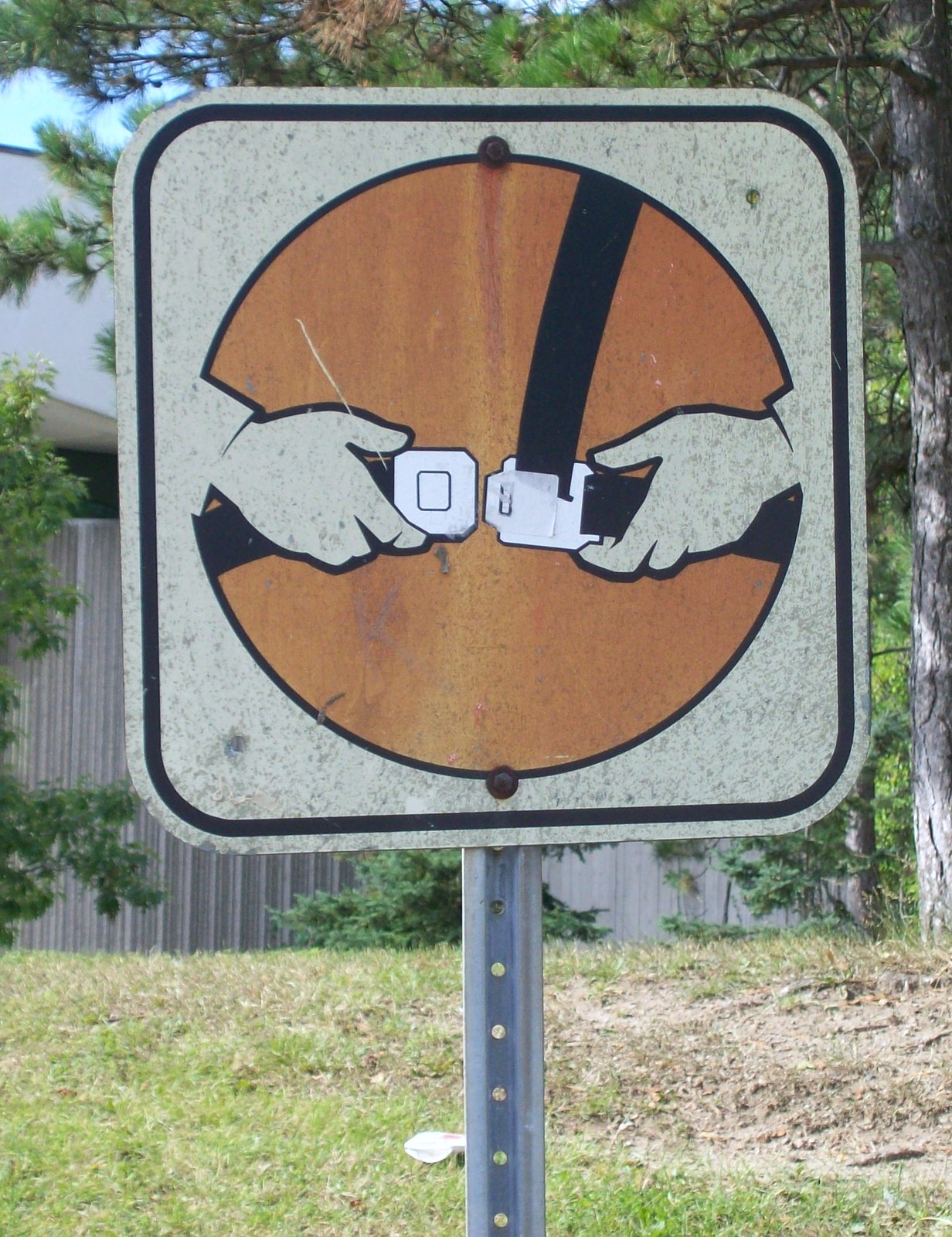A white, square sign with a black border stands outdoors, mounted on a metal pole with holes drilled into it. Central to the sign is a cartoon image depicting two hands fastening a seat belt, similar to those found in cars or airplanes. The person in the cartoon is dressed in orange-colored clothing. The sign is set against a picturesque backdrop featuring a grassy hill, a wooden fence, and a tree, emphasizing the importance of wearing a seat belt for safety.